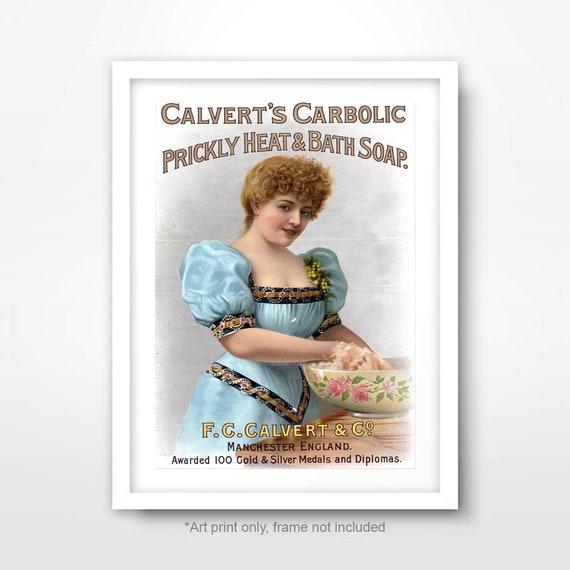This art print advertisement depicts a vintage promotion for Calvert's Carbolic Prickly Heat and Bath Soap. At the top, the text "Calvert's Carbolic Prickly Heat and Bath Soap" appears in brown-capped font. The focal point is a detailed illustration of a young, slightly buxom, possibly Victorian-era woman with short, curly reddish-strawberry blonde hair. Her complexion is fair with rosy cheeks and crimson lips, and she smiles warmly as she looks out from the picture. She is adorned in an exquisite baby blue, somewhat low-cut dress with poofy shoulder pieces, elaborate royal blue and gold trimmings, and a floral brooch. The woman’s hands, immersed in a ceramic bowl decorated with pink flowers and green leaves, are covered in foamy soap bubbles, suggesting she's washing her hands. Below this charming scene, the text reads, "F.C. Calvert & Co., Manchester, England, awarded 100 gold and silver medals and diplomas," signifying the product's accolades. It’s important to note the fine print at the bottom stating, "Art Print Only, Frame Not Included." The background is clear white, accentuating the artwork for a clean presentation.